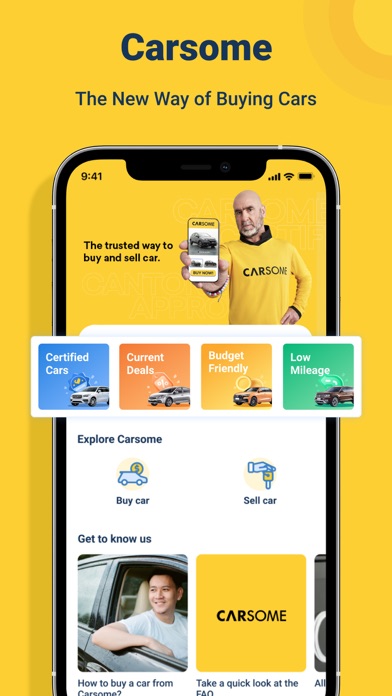**Detailed Caption:**

This image is a screenshot of a Carsome advertisement with a vibrant background. The top section of the background is a bright orange, featuring dark blue text that reads "Carsome." Below this main title, in smaller dark blue font, is the slogan: "The new way of buying cars." 

In the center of the image, there is a graphic of a smartphone with black bezels. The upper left corner of the smartphone screen displays the time as "9:41," and the upper right corner has icons for mobile signal, Wi-Fi, and battery status. 

Beneath these icons, the smartphone screen mirrors the advertisement's orange background. In the same dark blue font, it reads: "The trusted way to buy and sell a car." To the right of this text, there is a photo of a white, bald man with a gray goatee. He is wearing an orange sweatshirt with the "Carsome" logo in dark blue font and has a dark blue collar. The man is holding up a smartphone displaying this exact same screen in a recursive effect.

At the bottom, the advertisement features a white rectangle housing four smaller icons. Starting from the left, the first icon is a blue square with white text that says "Certified Cars" accompanied by a car image. To its right is an orange square with white text "Current Deals" also featuring a car image.

This well-designed advertisement effectively blends text, colors, and graphics to convey the company's innovative approach to buying and selling cars.